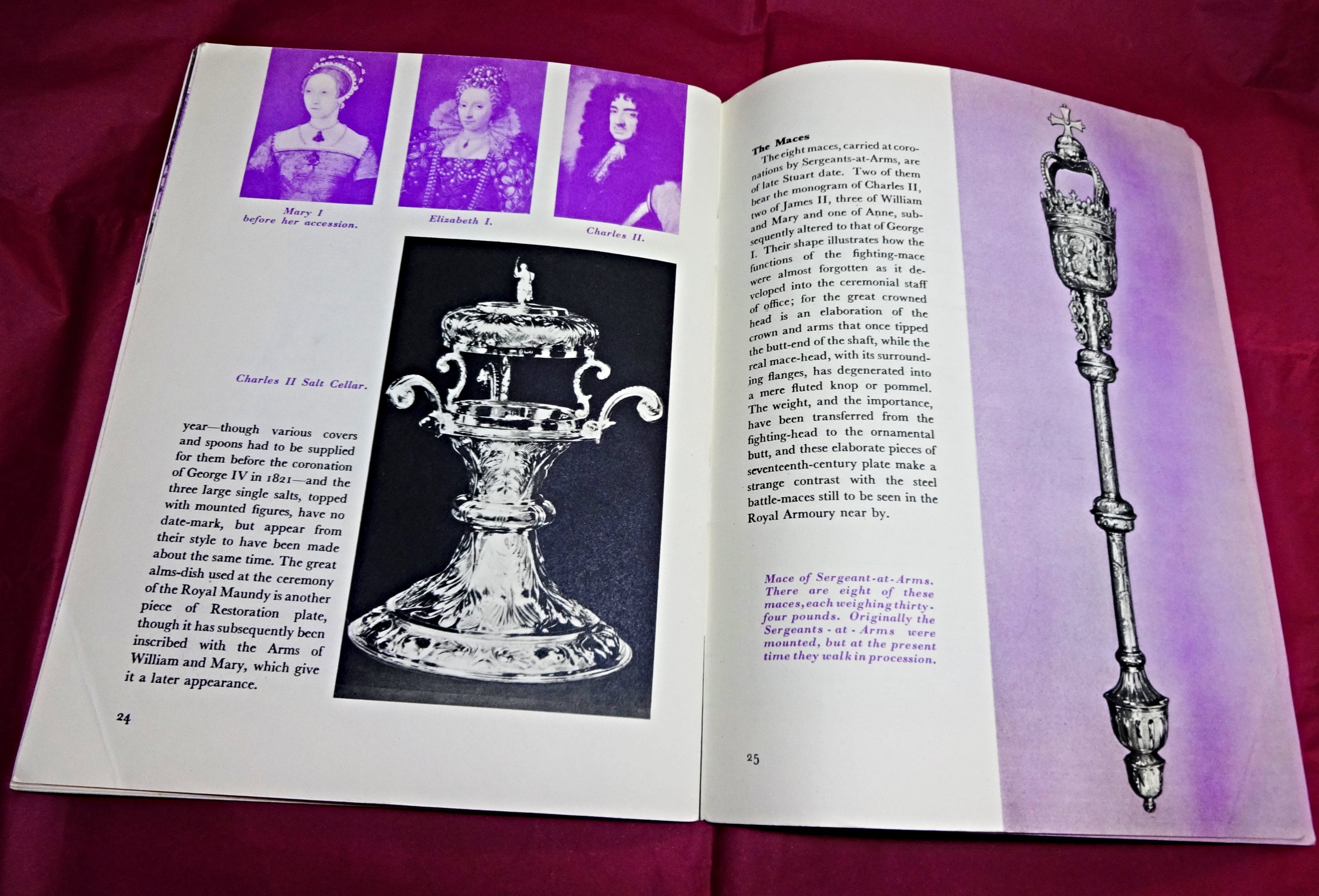This color photograph features an open magazine or pamphlet laid against a dark wine red tablecloth background. The visible pages are numbered 24 and 25. On the left page, the top section showcases purple-tinted portraits of Mary I, Elizabeth I, and Charles II. Beneath these portraits, the text "Charles II Salt Cellar" appears, accompanied by a paragraph of black text. An image of the salt cellar, which resembles an ornate chalice, is also present. The right page contains an article titled "The Maces," featuring another paragraph of black text. Adjacent to this text is an image of a ceremonial mace, depicted over a purple background. The pages are bordered in purple, adding to the regal theme of the article about the British monarchy.